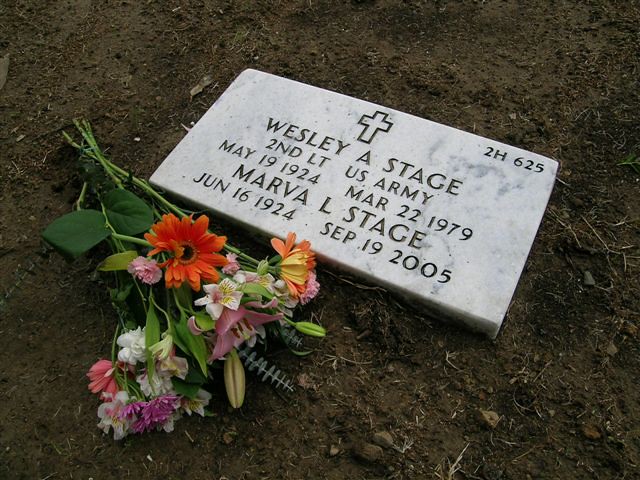This image is a detailed close-up of a rectangular marble headstone plaque resting on dark, freshly dug dirt. The headstone, which is flat to the ground, is slightly tilted to the viewer's right. Engraved in the upper right-hand corner of the plaque is "2H 625." Centrally positioned on the plaque is an engraved cross. Below the cross, the inscription reads, "Wesley A. Stage, 2nd LT U.S. Army, May 19, 1924 - March 22, 1979." Underneath, it also commemorates "Marva L. Stage, June 16, 1924 - September 19, 2005." On the bottom left side of the plaque, there is a bunched bouquet of flowers, featuring orange, white, and pink blooms alongside green stems. The surrounding area is primarily dark brown dirt, interspersed with some small rocks and fragmented roots.